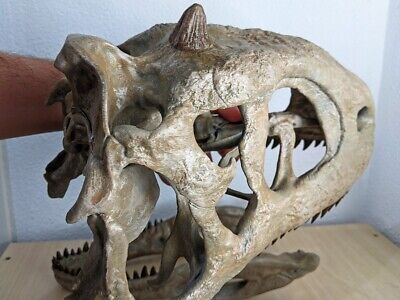The image showcases a close-up, well-preserved skull, likely of a prehistoric creature, possibly a dinosaur or an ancient tortoise, displayed in a light wooden tray against a faint background of a dark white to light blue wall. The elongated skull, featuring an oval shape with a pronounced posterior and a flattened nose region, suggests an aquatic or semi-aquatic animal. The jaw, partially open, reveals rows of sharp, small black teeth, hinting at a carnivorous diet. Eye sockets and facial features are distinctly identifiable. A prominent horn sits atop the skull, and the overall coloration is a blend of gray with some worn brownish-tan accents, indicating its age. An outstretched arm of a man holding up the skull is visible in the background, emphasizing its display quality, much akin to a museum exhibit.